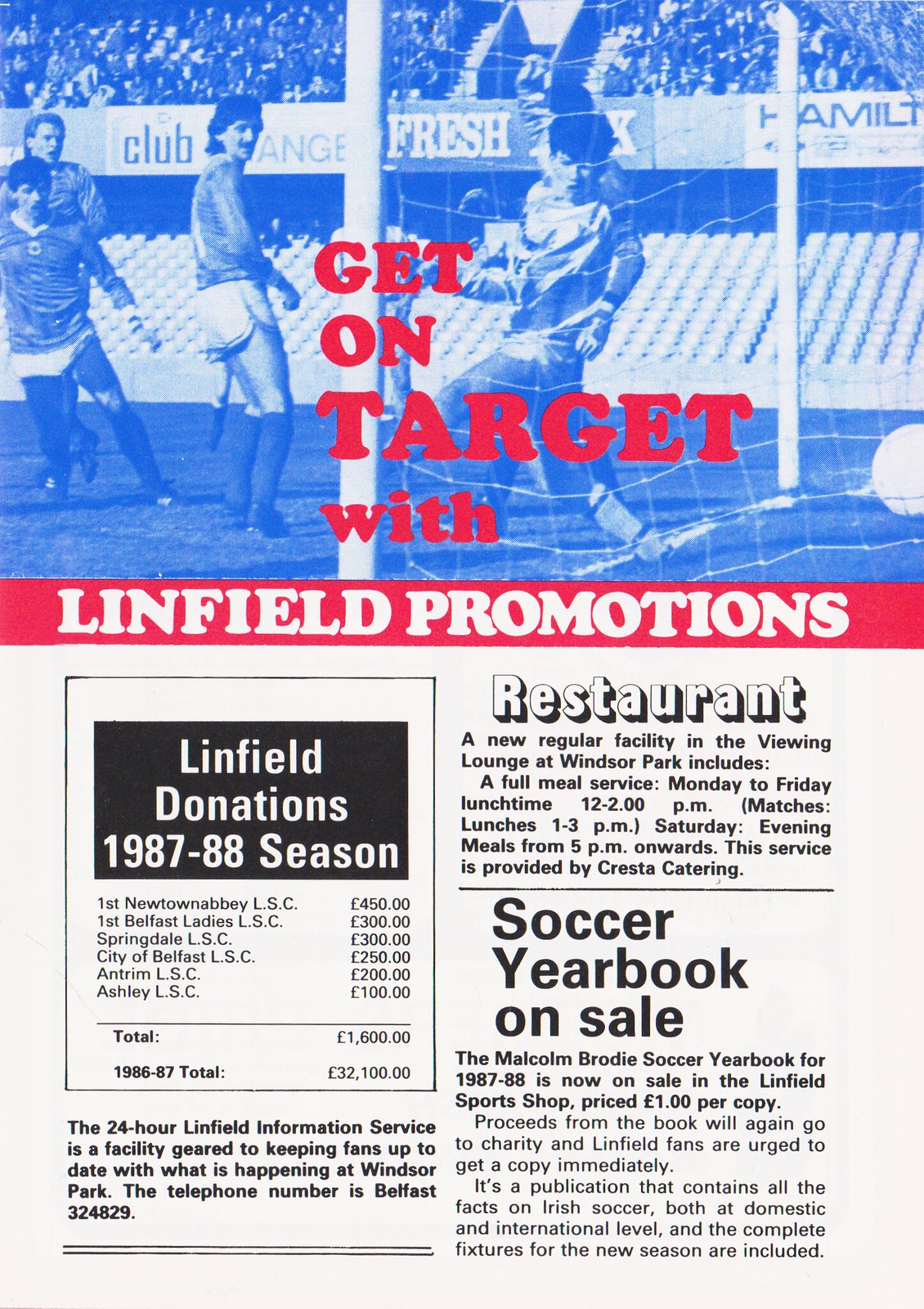This page from a game day program or magazine serves as an old advertisement for Linfield Sports Shop. The top half is dominated by a blue and white photograph of four men playing soccer, with stands full of audience behind them. Overlaying this image is red text reading, "Get on target with…" and then beneath it, in a red banner with white text, "Linfield Promotions." Together, it reads, "Get on target with Linfield Promotions." 

Below the image, on the left side, a black square outlines a list titled "Linfield Donations, 1987-88 season." It's detailed with various contributions:

- First Newtown Abbey's LSC: £450
- First Belfast Lady's LSC: £300
- Springfield LSC: £300
- City of Belfast LSC: £250
- Antrim LSC: £200
- Ashley LSC: £100

Total donations amount to £1,600, with an impressive total from the previous season (1986-87) of £32,100. Adjacent to this, a section details a new restaurant at Windsor Park. Operated by Crested Catering, it offers a full meal service Monday to Friday from 12-2 p.m., and match-day lunches from 1-3 p.m. Saturday evening meals start from 5 p.m. onwards.

A section beneath the restaurant notice announces the "Soccer Yearbook On Sale." The Malcolm Bronte Soccer Yearbook for the 1987-88 season, priced at 1 euro per copy, is available at the Linfield Sports Shop. Proceeds go to charity, and fans are encouraged to purchase a copy. The publication includes comprehensive information on Irish soccer at both domestic and international levels, as well as the complete fixtures for the new season.